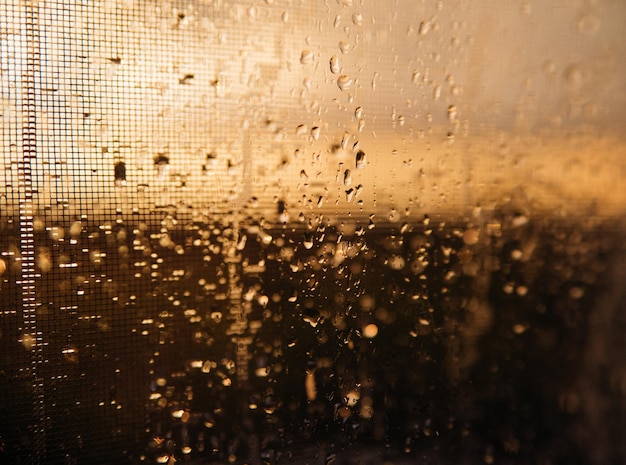The photograph presents a moody, close-up view of a rain-soaked window screen, with an interplay of focus that creates a captivating depth. Dominated by droplets of water, the image captures the essence of a rainy day. The left side of the photograph distinctly reveals the mesh of the window screen, while the right side transitions into a blur, emphasizing the central focus on the droplets. The background exhibits a gradient from dark to light, with dark tones at the bottom possibly representing the ground and lighter hues at the top suggesting a grey, overcast sky. The overall sepia-golden tone imbues the scene with a warm, nostalgic feel, enhancing the sense of motion as if the droplets are gently sliding down the screen. The detail in the middle of the photo, particularly the rain droplets, stands out clearly against the soft, ambiguous backdrop, creating a serene and contemplative visual experience.